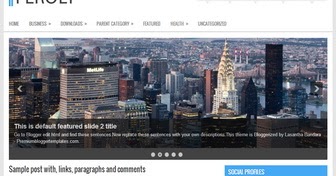This image is a blurry screenshot from an unidentified website, partially cropped to the extent that the site's full title is obscured. The top-left corner shows a fragment of the title in large, bold font alongside blue stripes, which may likely represent the site's logo. Against a general white background, there's a navigation bar visible, with tabs labeled "Home," "Business," and "Features," among potentially others that are difficult to discern due to the image quality.

Beneath the navigation bar, there is a prominent rectangular cover image displaying a landscape of New York City with numerous skyscrapers. Overlaid on this cover photo, towards the bottom, there is a semi-transparent black caption stating "This is default feature slide to title," with additional, smaller text below it that is indistinguishable. 

Centered at the bottom of the image, five circles denote the pagination of the gallery, with the second circle highlighted to indicate the current page. Flanking the image, arrows on the left and right edges hint at navigation options for traversing through the gallery.

Further down the page, the bottom-left corner mentions "Sample Post with Links, Paragraphs, and Comments," suggesting a sample post content area. Meanwhile, on the bottom right, there is a blue section labeled "Social Profiles," perhaps for user interaction or connectivity options on social media.